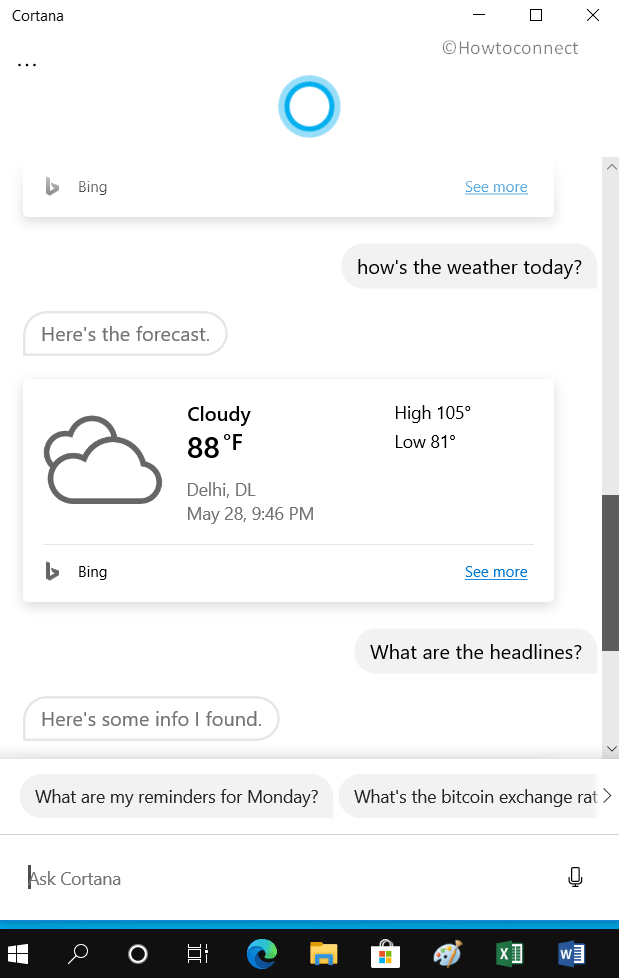The image is a detailed screenshot of the Cortana virtual assistant on a Windows 10 operating system. The screenshot bears a watermark "copyright how to connect," written as one word. The desktop displays a conversation with Cortana, where the user inquires about the weather with the query, "How's the weather today?" Cortana responds with, "Here's the forecast: Cloudy, 88 degrees. Delhi, D.O. May 28, 9:46 p.m. Hi: 105 degrees. Low: 81 degrees. From Bing. See more.” 

Following the weather inquiry, the user asks, "What are the headlines?" Cortana replies, "Here’s some info I found," but the rest of the conversation is truncated, cutting off further details.

At the bottom of the Cortana interface, the text entry box prompts the user with the message, "Ask Cortana." Above this box, suggested questions include, "What are the reminders for Monday?" and "What's the Bitcoin exchange rate?"

The Windows taskbar is visible, featuring several icons from left to right: the Windows Start button, search button, Cortana icon, Timeline view, Microsoft Edge, File Explorer, Microsoft Store, Microsoft Paint, Excel, and Microsoft Word.